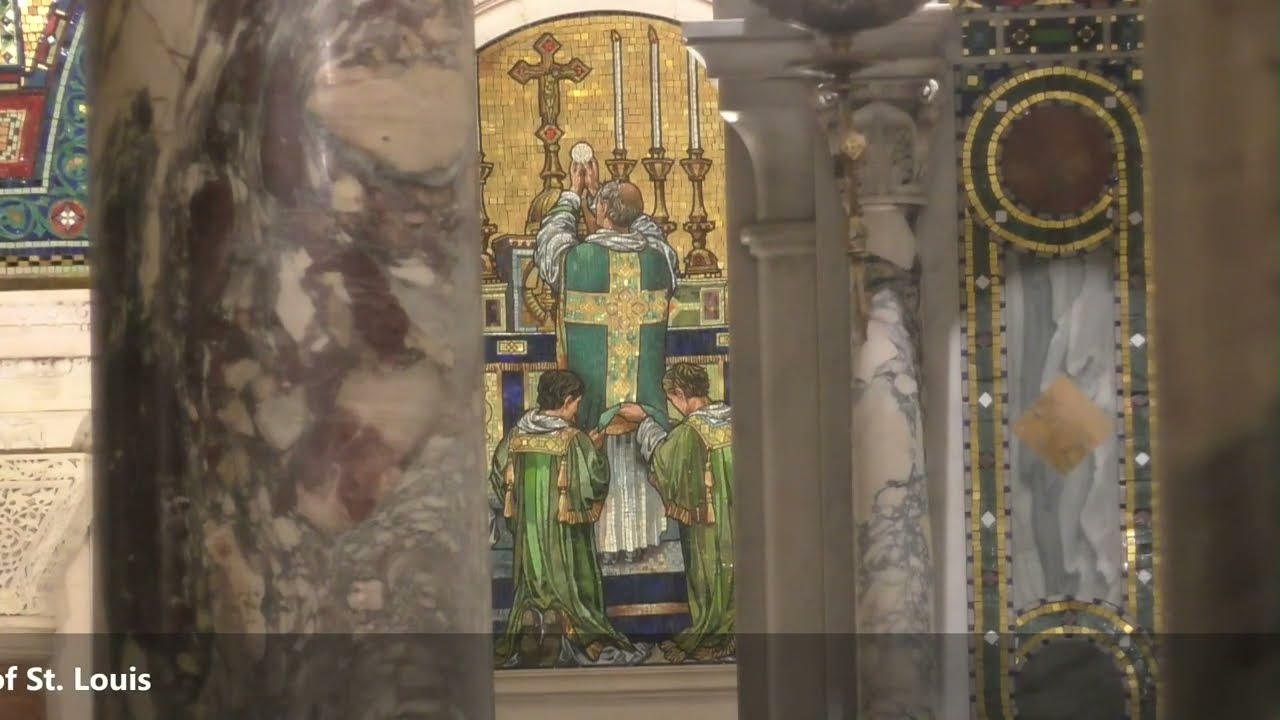The image captures a highly detailed scene within a religious setting, likely within a church, featuring vibrant colors and intricate decorations. Dominating the center is a two-dimensional, 10th-century styled mosaic that depicts a ceremonial scene. In this mosaic, a priest, clad in a flowing robe with a dark green top adorned with a yellow cross, is depicted with his hands raised above his head, holding a circular object, suggestive of the Eucharist. Flanking the priest are two youthful altar boys, shown assisting with the ceremony. The background of the mosaic is rich in religious symbolism, including a crucifix and three tall candles ensconced in elaborate bronze stands to the right.

The foreground of the scene showcases large marble-like columns, with a prominent one on the left and additional smaller columns on the right side of the image. The pillars frame the sacred imagery and add a grand architectural element to the setting. The left side of the image is partially obscured by these columns, but small portions of a circular mosaic pattern and more of the church interior are visible, reflecting white walls and additional mosaic artwork.

A fragment of text is visible at the bottom left, reading "of St. Louis," though it is incomplete. The church’s interior is illuminated with ample light that enhances the vivid colors which range from white, burgundy, yellow, green, gold, black, to red, contributing to the overall clarity and brightness of the scene. Whether the image represents a model or a life-size view remains indiscernible from the current perspective, yet it provides a rich, detailed glimpse into the religious and artistic heritage depicted.